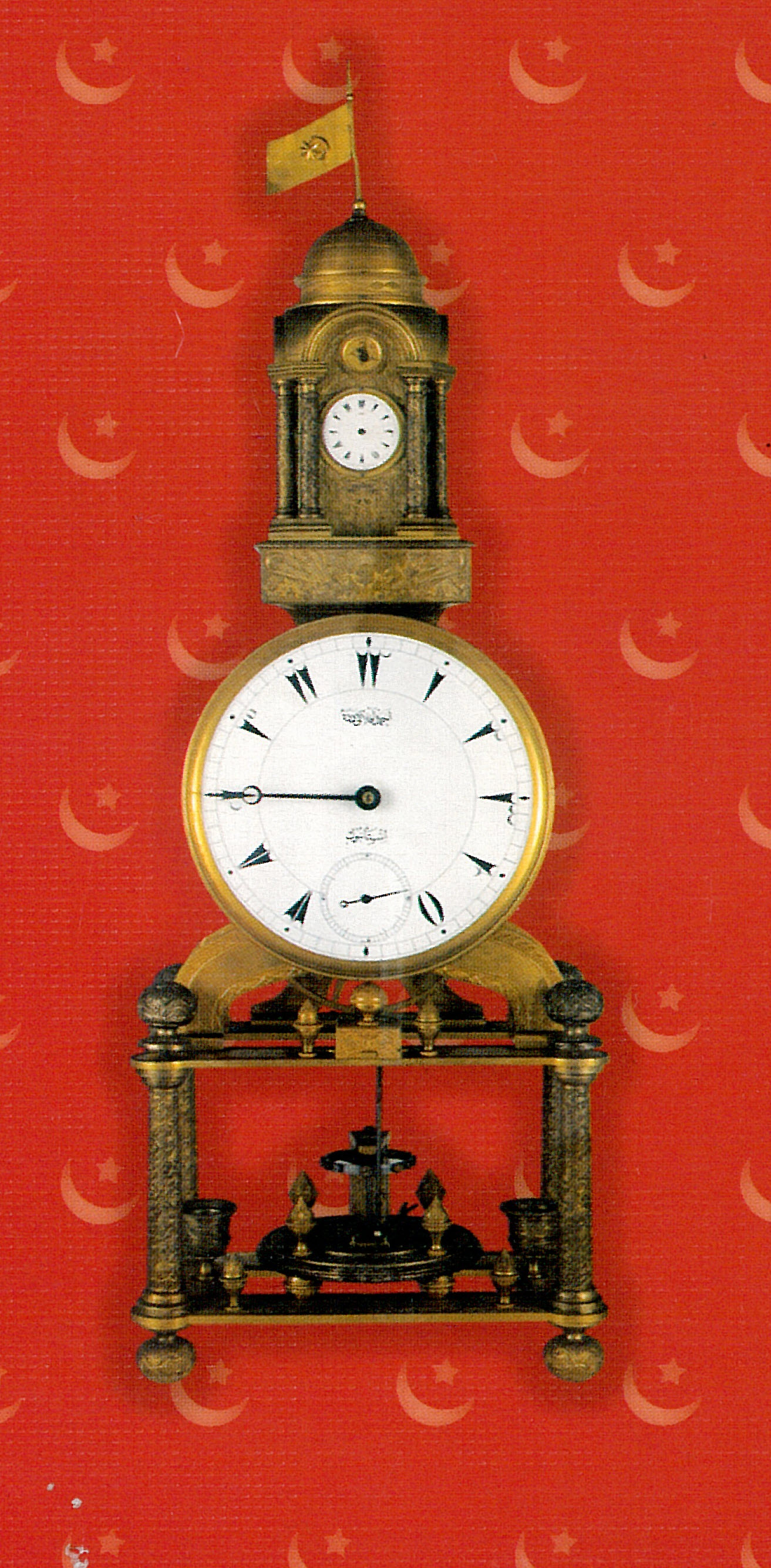The image depicts a highly ornate, vintage clock that appears to be made primarily of brass. The clock stands atop an elaborate pedestal supported by four brass columns with intricate etching. The columns rest on rounded oval bases, framing a visible mechanism—a dark bronze disc with protrusions—nestled between them. The clock has a white face encircled by a brass frame, featuring unconventional hour markers, with the 12 indicated by two triangles and other positions marked by symbols and tick marks of varying thickness. 

Above the main clock face is a smaller clock face integrated within a dome structure, topped with a brass flag bearing a starburst, pointing left. The clock features two sets of hands; one on the smaller face and another on the larger face below it. Notably, the hour and minute hands on the primary face originate from different points. At the base, a rotating pendulum is plainly visible, adding to the intricacy of the mechanism.

The backdrop is vibrant red with a textured, cross-hatched pattern embellished with repeated crescent moons containing stars, heightening the overall visual appeal. The detailed craftsmanship and unique design elements strongly suggest the image might be a photorealistic rendering or an AI-generated illustration.